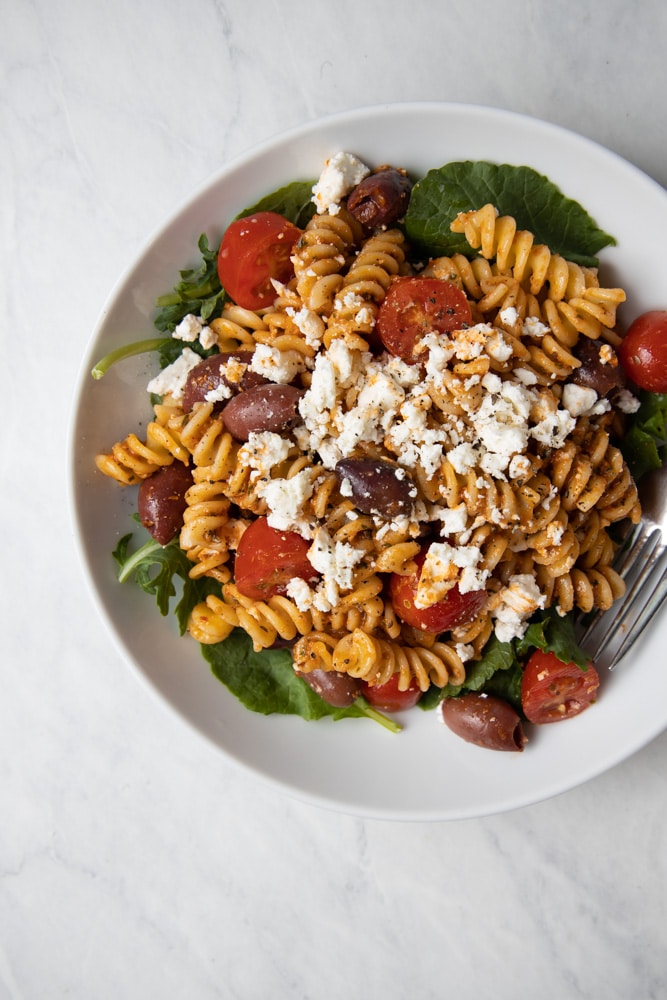This professional photograph showcases a vibrant pasta salad meticulously presented in a white round plate. The plate rests on a pristine white marble countertop streaked with elegant gray veins, captured from a top-down perspective. The base of the salad is a bed of fresh spinach leaves, layered with tan-colored rotini pasta. Interspersed among the pasta are halved red cherry tomatoes and flavorful kalamata olives. The ensemble is crowned with crumbles of feta cheese and a light sprinkling of cracked black pepper, possibly complemented by a drizzle of olive oil. A silver fork is elegantly placed in the bottom right-hand corner of the plate, inviting the viewer to savor the dish. This colorful and appetizing pasta salad, featuring vibrant reds, oranges, and greens, is a delightful blend of Italian and Mediterranean elements, offering a feast for both the eyes and the palate.